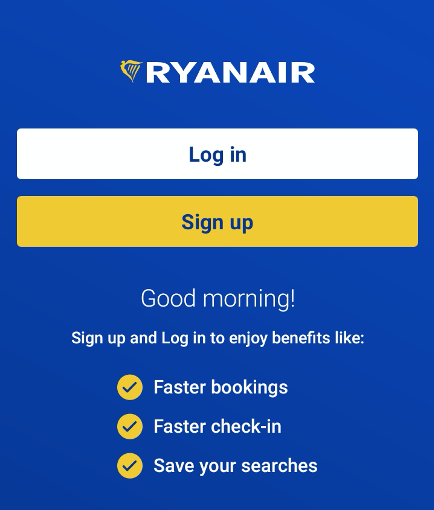This is a screenshot of the Ryanair website, showcasing a bright blue background with a clean and modern layout. At the top center of the page, the Ryanair logo is prominently displayed in white, accompanied by a smaller yellow harpsichord symbol to the left. In the same header section, a white "Log In" button is visible, seamlessly blending with the background. Directly below it, a yellow "Sign Up" button appears, featuring white text in a slightly thinner font.

The main content area greets users with the message "Good Morning," followed by an invitation to "Sign up and log in to enjoy benefits like:" Below this text, there are three feature highlights, each accompanied by a blue check mark that acts as a bullet point. These features are listed as:
1. Faster bookings.
2. Faster check-in.
3. Save your searches.

The overall design of the website is intuitive and user-friendly, with clear calls to action and a cohesive color scheme that makes navigation straightforward.